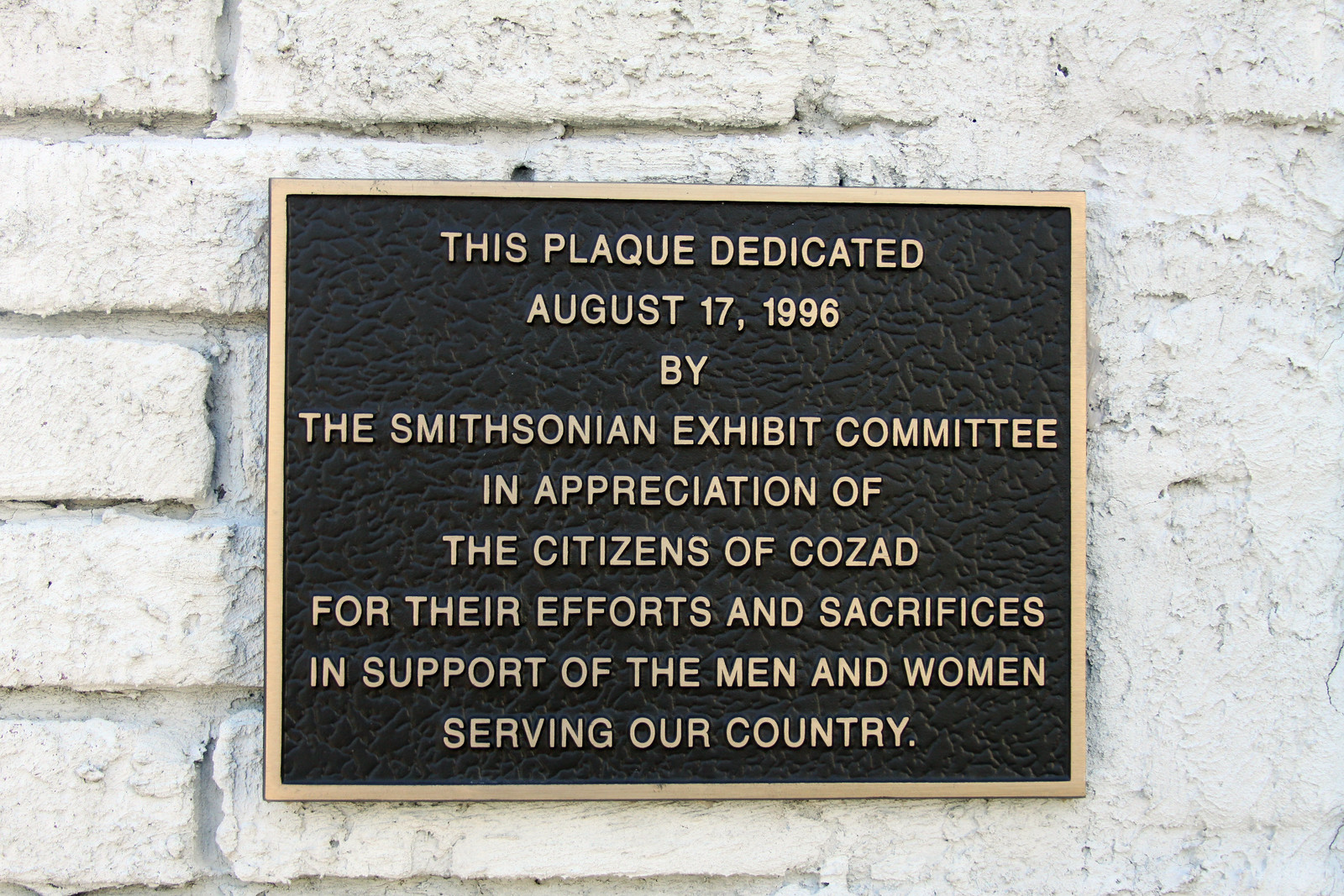In this image, a metal plaque is prominently displayed against a white-painted brick wall, positioned centrally within the frame. The plaque features a bold, black background with a wavy, leather-like texture and is bordered by a gold frame. The text on the plaque, also in a matching gold color, reads: "This plaque dedicated August 17, 1996 by the Smithsonian Exhibit Committee in appreciation of the citizens of Kozad for their efforts and sacrifices in support of the men and women serving our country." This outdoor setting likely places the plaque on the side of a building or monument, serving as a memorial tribute.